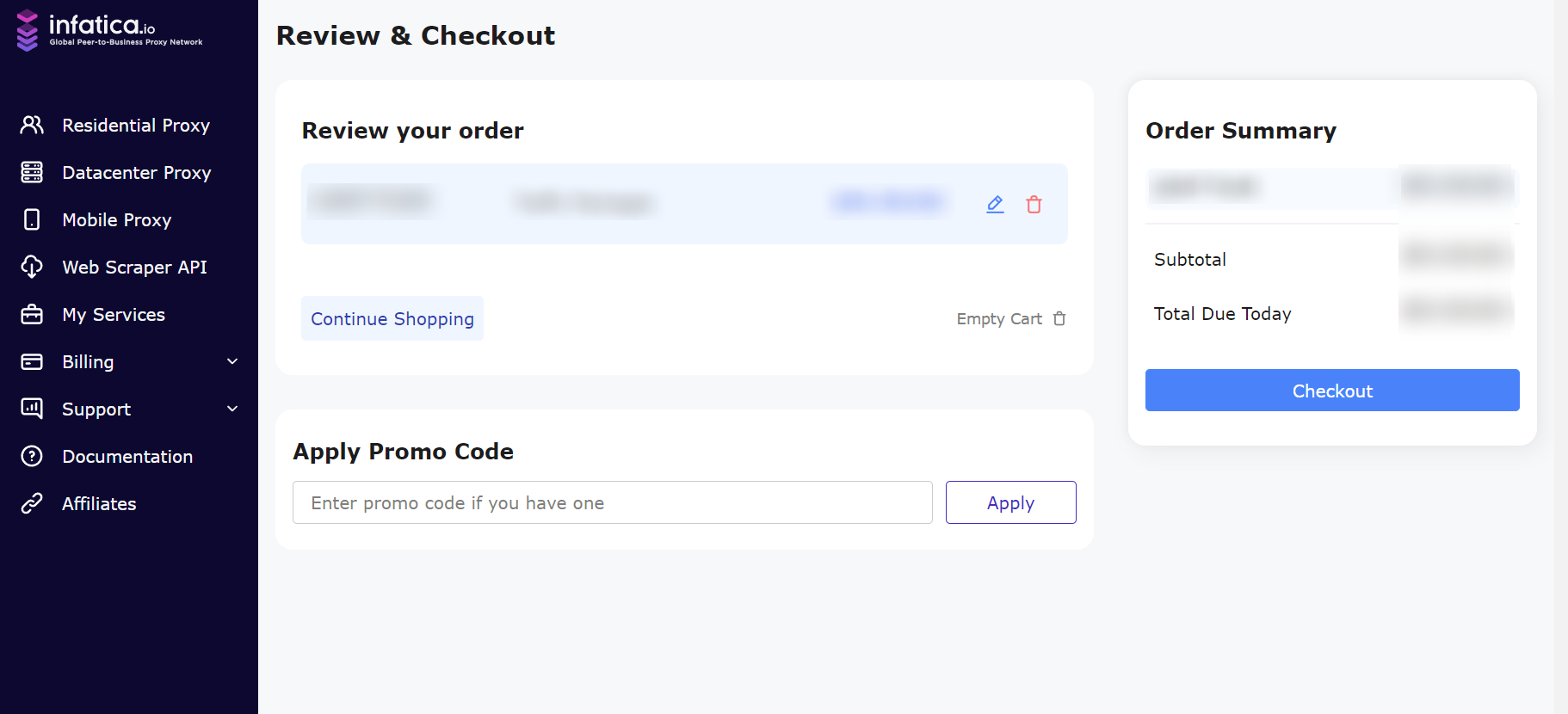The image depicts a detailed screenshot of the checkout page for an order placed on Infatica.io, a website indicated by a navvy blue border running vertically along the left side of the image. At the top of this left-side border, the company’s logo "Infatica.io" is prominently displayed, featuring the name in white block letters and a distinctive purple and red stacked icon resembling a computerized graphic.

Immediately below the logo, a vertical menu is organized into several categories each accompanied by specific icons: 
- "Residential Proxy," "Data Center Proxy," and "Mobile Proxy" options each represented by corresponding icons.
- "Web Scraper API," "My Services," "Billing," "Support," "Documentation," and "Affiliates," each signified with unique icons like a download arrow, shopping bag, and credit card.

The right section of the screenshot, bordered in gray, centers on the "Review and Checkout" process. The section first instructs users to "Review your order." A blue box occupying this section is partially blurred, likely to obscure sensitive information, and includes a pencil icon for editing and a trash can for removing items.

Below this, options for "Continue Shopping" and "Apply Promo Code" are available. The promo code section features a field labeled "Enter Promo Code if you have one," beside an "Apply" button.
 
To the far right of this gray-bordered section, we find the "Order Summary," which clearly displays "Subtotal," "Total Due Today," and a prominent "Checkout" button for finalizing the purchase.